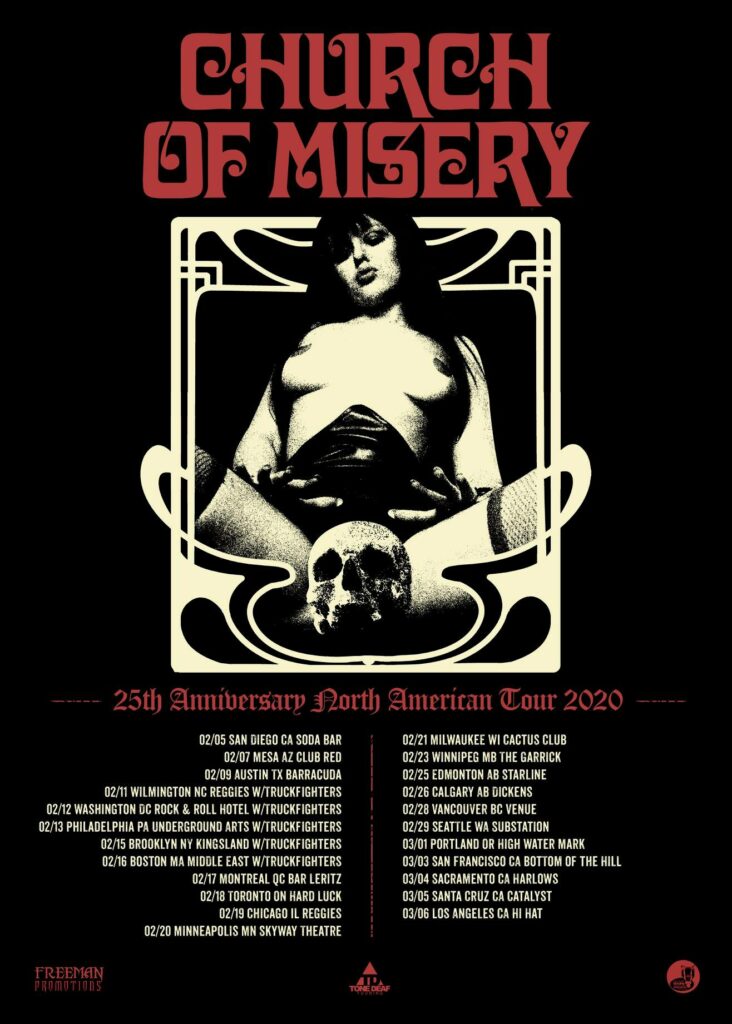The image is a poster commemorating or advertising the 25th Anniversary North American Tour 2020 for the band "Church of Misery." The background is entirely black. At the top of the poster, in red, all-capital letters, it says "CHURCH." Below that, also in large red capital letters, it says "OF MISERY," which is centered. 

In the middle of the poster, there is a cream-colored frame surrounding an image of a topless woman with long black hair. She is slightly leaning back with her legs crisscrossed in front of her, and she appears to be wearing fishnet stockings. Strategically placed to cover her crotch is a human skull. 

Below this framed image, in red calligraphy, the text reads "25th ANNIVERSARY NORTH AMERICAN TOUR 2020." Further below, a list of various cities, dates, and venues where the band will be performing is displayed. Some noted locations include San Diego, California (Soda Bar); Mason, California (Club Red); Austin (Barracuda); and Wilmington, North Carolina (Regals with Truck Fighters). 

Towards the bottom left of the poster, "Freedom Promotions" is printed in red, while in the middle, it says "Tefdo, Teftone Death," adding further artistic flair to the design. Overall, the poster has an evocative and dark aesthetic, fitting the band's image and the announcement of their tour.